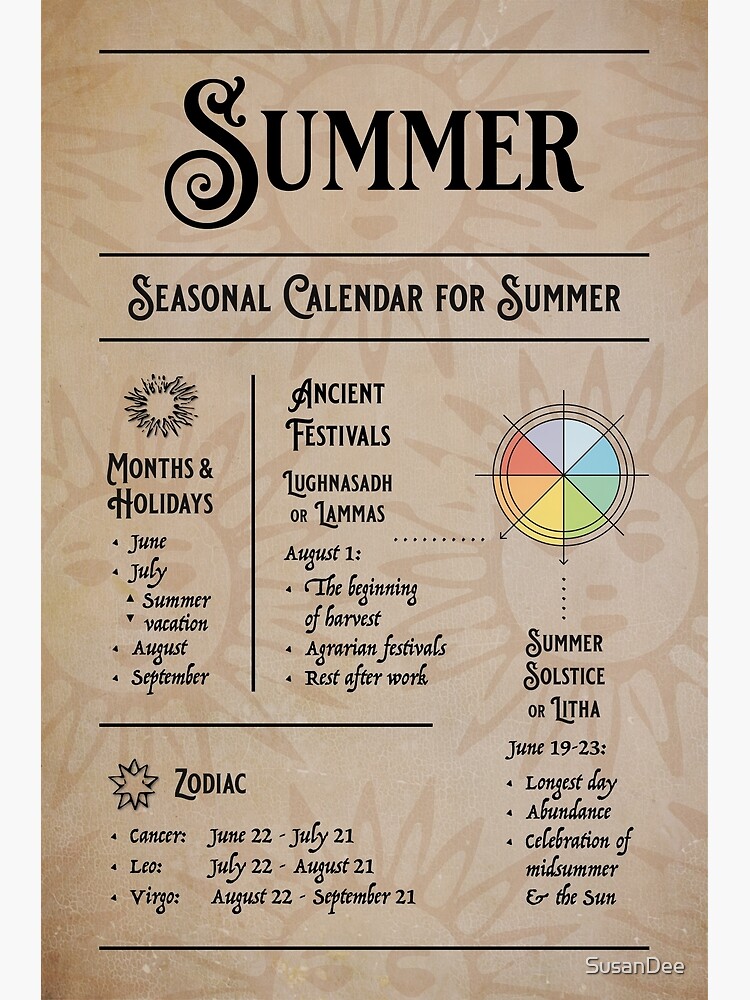The image is a brochure or informational page with a brownish-beige background, featuring a faded, neutral-faced sun with pointy rays imprinted on the paper. Across the top in large, stylized black lettering is the word "SUMMER," with extra curves emphasizing the "S." Beneath this are two horizontal black lines, between which it reads "SEASONAL CALENDAR FOR SUMMER." The content is divided into sections: 

On the left side, it lists "MONTHS AND HOLIDAYS" in capitalized letters, followed by bullet points for "June," "July" (noted with a summer vacation symbol), "August," and "September." 

In the middle section, titled "ANCIENT FESTIVALS," it mentions "Lughnasadh or Lammas" on "August 1st," described as "the beginning of harvest," with additional bullet points for "agrarian festivals" and "rest after work." 

On the right side, there's a colorful pinwheel divided into rainbow segments, symbolizing various phases related to the summer period. Below this image, it states "SUMMER SOLSTICE OR LITHA, JUNE 19–23," highlighting it as "the longest day" and a "celebration of midsummer and the sun." 

At the bottom left section, it lists zodiac signs "CANCER," "LEO," and "VIRGO," along with their respective dates. The detailed layout and comprehensive information make this brochure a visually distinctive and informative guide for the summer season.